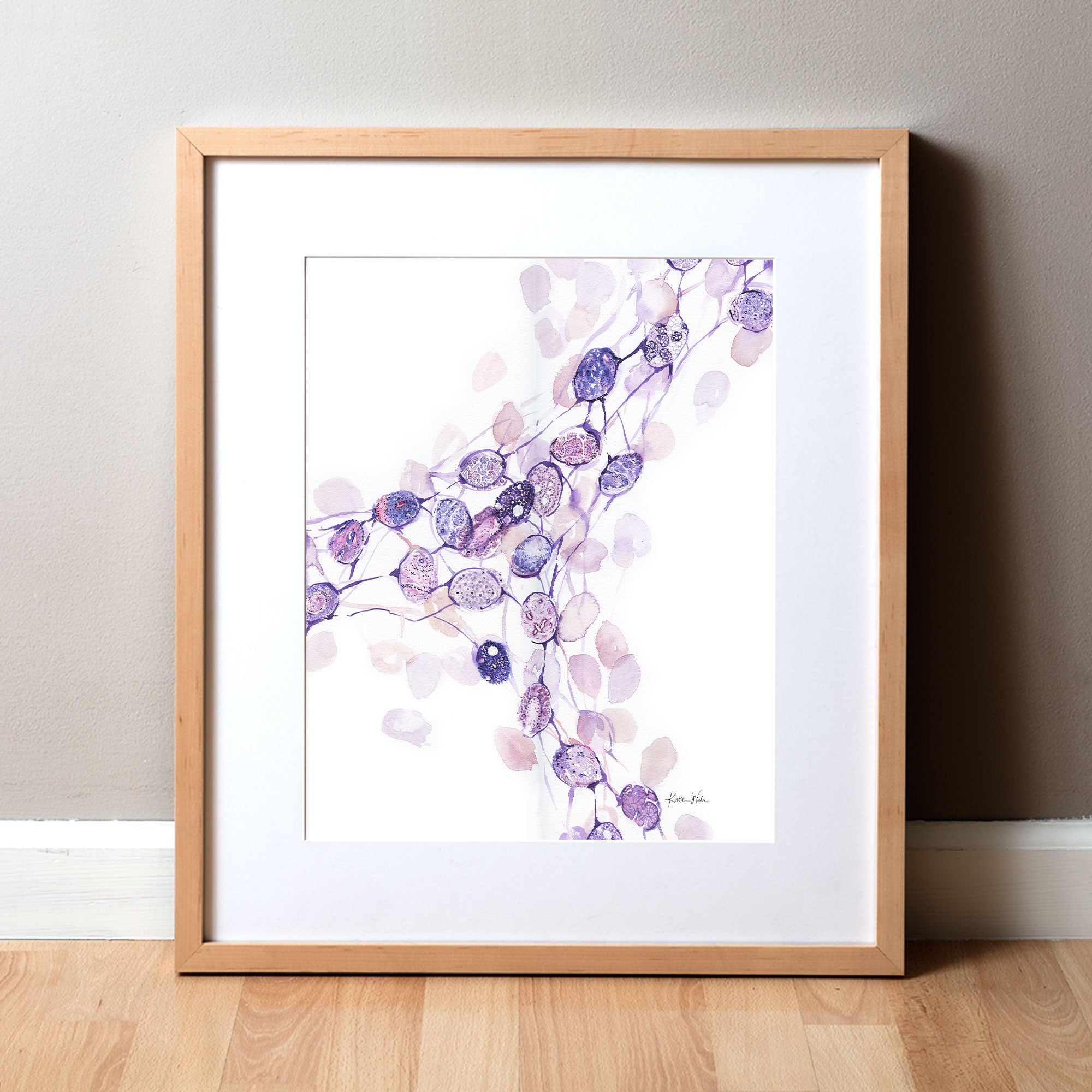This image is a stock photo showcasing a framed print of what appears to be either a nature or biology-themed artwork. The artwork features delicate, oval-shaped objects reminiscent of microorganisms or plant leaves, primarily in shades of pink, lilac, purple, and peach. These objects are intricately connected by fine lines, forming a T or Y shape, branching out from the lower left corner and splitting open towards the top. Some of the objects are more prominent, while others are faded, offering a nuanced depth to the composition. Intricate patterns can be observed within each oval shape, adding to the complexity of the piece.

The print is signed in the lower right corner by an unreadable signature and is mounted on a white mat within a light brown, wooden frame. The entire framed artwork leans against a gray wall with white wainscoting and sits on a hardwood floor. The setting appears to be indoors, likely within a home, providing a serene and sophisticated backdrop to the unique and visually appealing print.